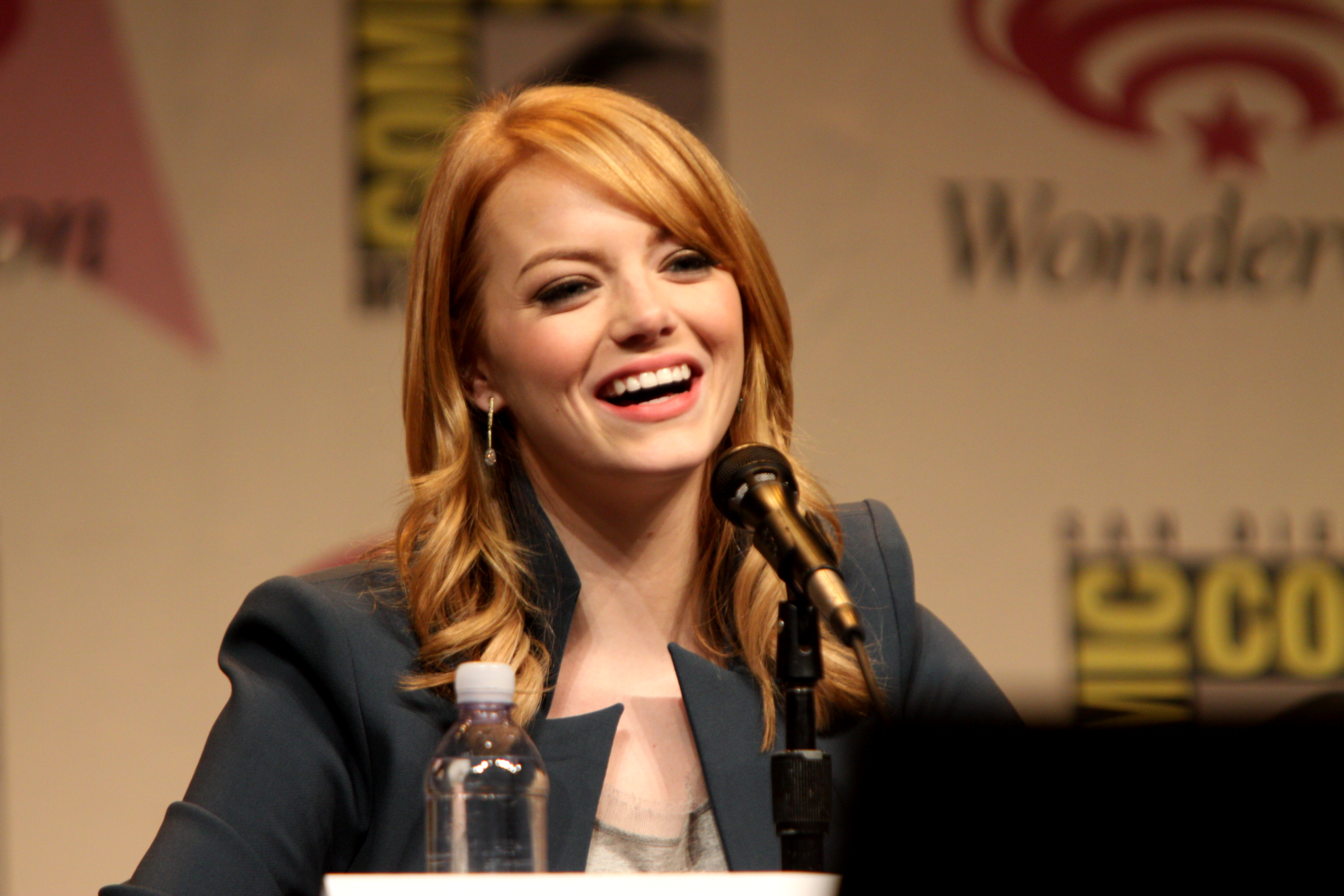The image depicts a young woman, an actor, with light blonde hair that has darker blonde streaks, cascading below her shoulders, and covering one ear while an earring is visible on the other. She is seated in front of a Comic-Con banner, which features repeated icons and an out-of-focus word "wonder" in the top right corner. Her head is slightly tilted to the left as she laughs heartily, revealing the top row of her teeth. She has pink lipstick and eyeshadow accentuating her cheerful expression. The woman is dressed in a dark gray jacket with a high collar, over a low-cut t-shirt. In front of her is a black microphone, and to its left, a clear water bottle with a white cap and the label removed. The background is predominantly white, indicating a stage setting.